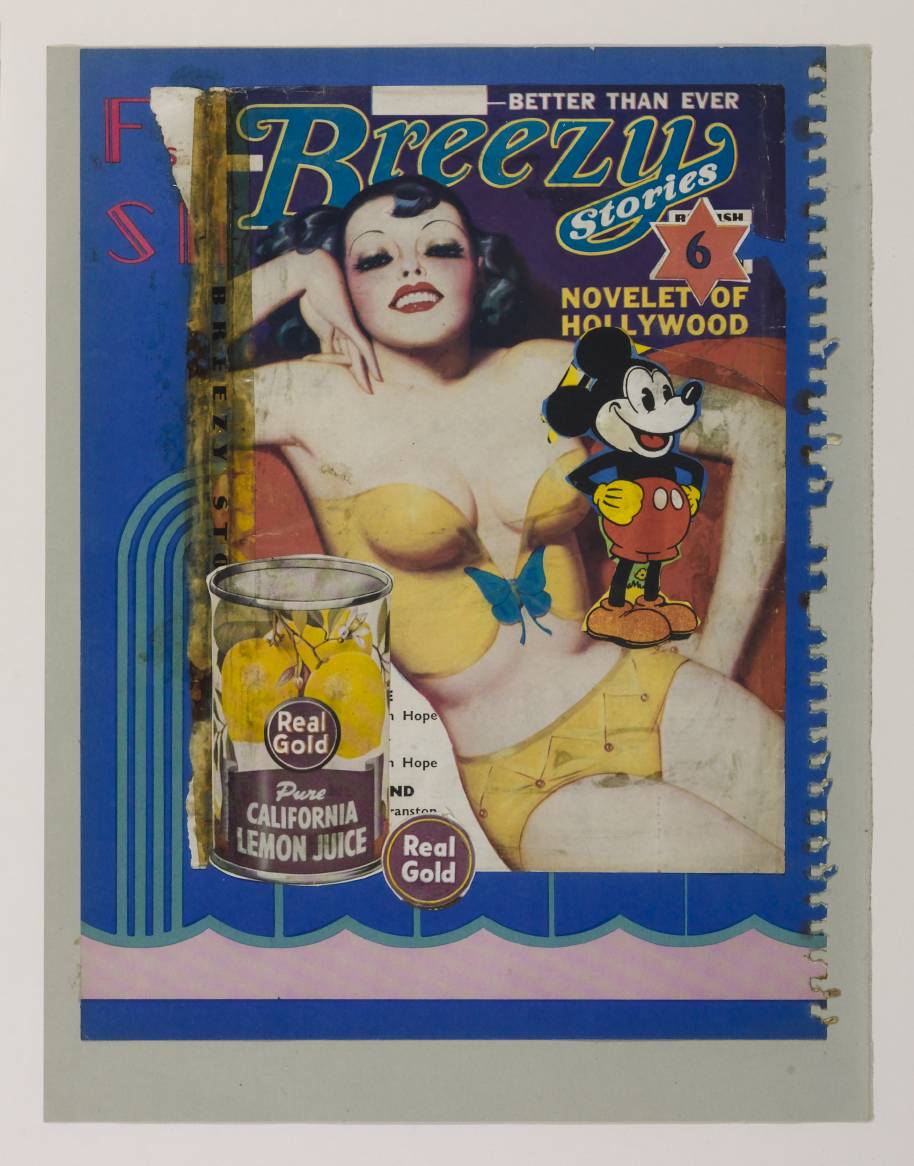The poster, designed to mimic a vintage magazine cover, features a distressed and frayed look, encapsulating a nostalgic Hollywood aesthetic. The background is a dark blue with a cream and light sage green border. At the top, bold white letters announce "Better Than Ever," followed by "Breezy Stories" in a bright turquoise, italicized font, encased in a yellow border. Below this, a red six-pointed star with a blue number six rests beside the phrase "Novelette of Hollywood" in gold text.

Central to the image is a reclining woman with a 1920s-style makeup, including thin eyebrows and bright red lips, and black hair. She wears a yellow bikini with a blue butterfly detail at the bustier-like top and yellow boy shorts. Her pose is relaxed, with one hand on her shoulder and the other on her hip, against a blue background. Superimposed over her hip stands a vintage cartoon Mickey Mouse, balancing and clutching his stomach. Overlapping this scene is an old-style label showing pears, labeled "Real Gold Pure California Lemon Juice."

The combination of eclectic elements – the nostalgic Mickey Mouse, the lemon juice can, and the vintage stylistic choices – contributes to a disjointed yet charming collage effect, highlighting the Hollywood allure of yesteryears.